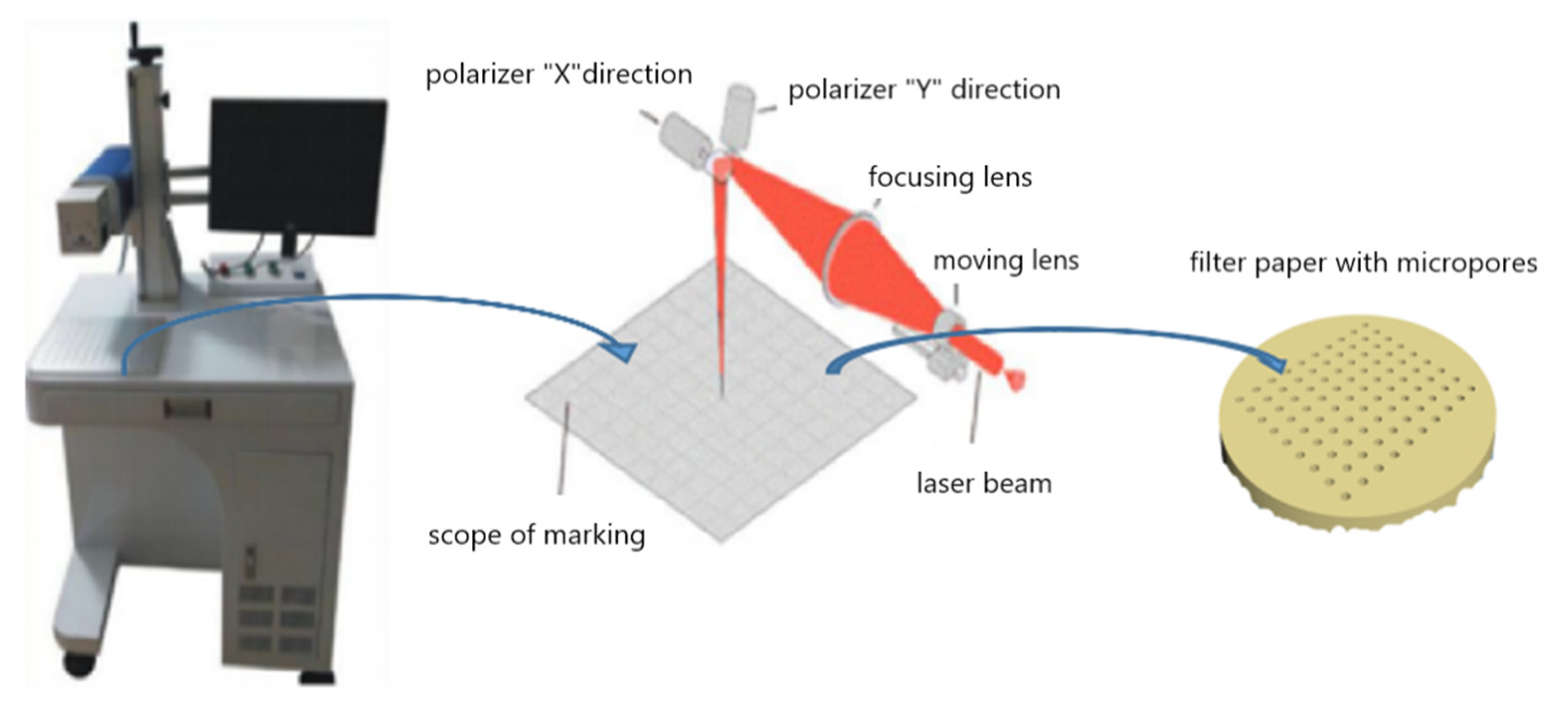The image showcases a detailed, instructive photo of a scientific microscope setup, typically found in technical or medical environments. On the left side, a table supports a sophisticated microscope apparatus connected to a computer monitor, which displays various components of the system. The center of the image focuses on the intricate details and labeling of the microscope's parts, illustrating the pathway and function of the device. Key features include a focusing lens, a moving lens, and a laser beam that highlight how the microscope is utilized. Labels indicate the polarizer X and Y directions, and further down, a filter paper with micropores is shown, used to observe objects underneath the microscope. The right side of the image presumably contains the filter paper, illustrating its placement and purpose within the scope. The overall setup appears mobile, possibly mounted on wheels for easy movement, and the entire assembly is meticulously detailed, breaking down the complex structure step-by-step.